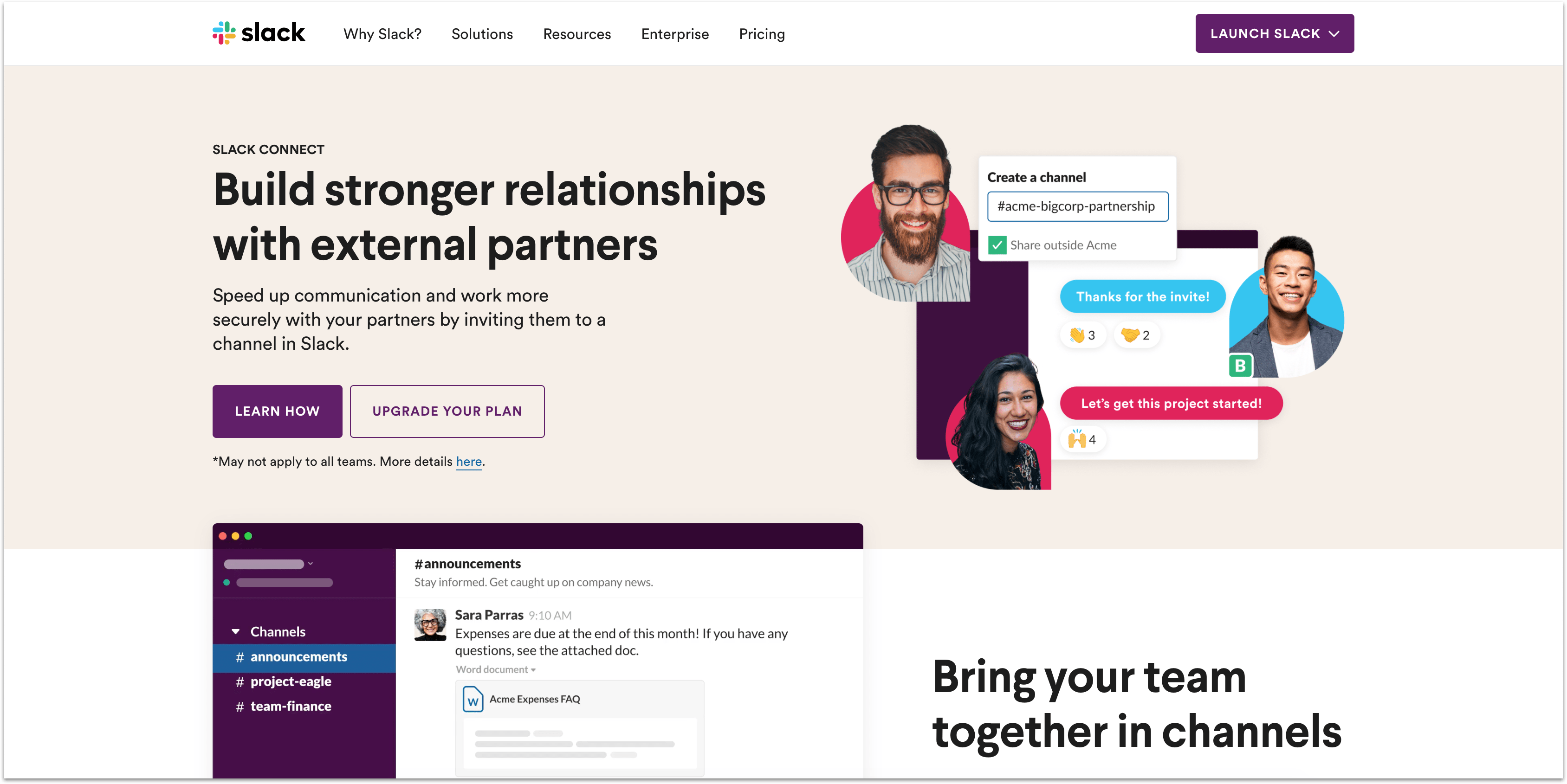The image depicts a screenshot from Slack's website. The word "slack" is prominently displayed in lowercase letters alongside a multicolored icon featuring teal, green, yellow, and red hues. At the top navigation bar, the options "Why Slack," "Solutions," "Resources," "Enterprise," and "Pricing" are listed. Towards the far right of this row, there’s a purplish button with the text "Launch Slack" in white.

The main section of the image has a tan background, while the bottom section transitions to a white background. In the tan area, the text reads "Slack Connect: Build stronger relationships with external partners. Speed up communication and work more securely with your partners by inviting them to a channel in Slack."

In the middle right area of the tan section, there is an illustration of three people. The top figure is a man with black glasses, a beard, and a mustache, all likely brown. Below him is a woman with long black hair. These figures appear to be engaging in communication, depicted through graphical elements. Additionally, there is another man shown within a blue speech bubble.